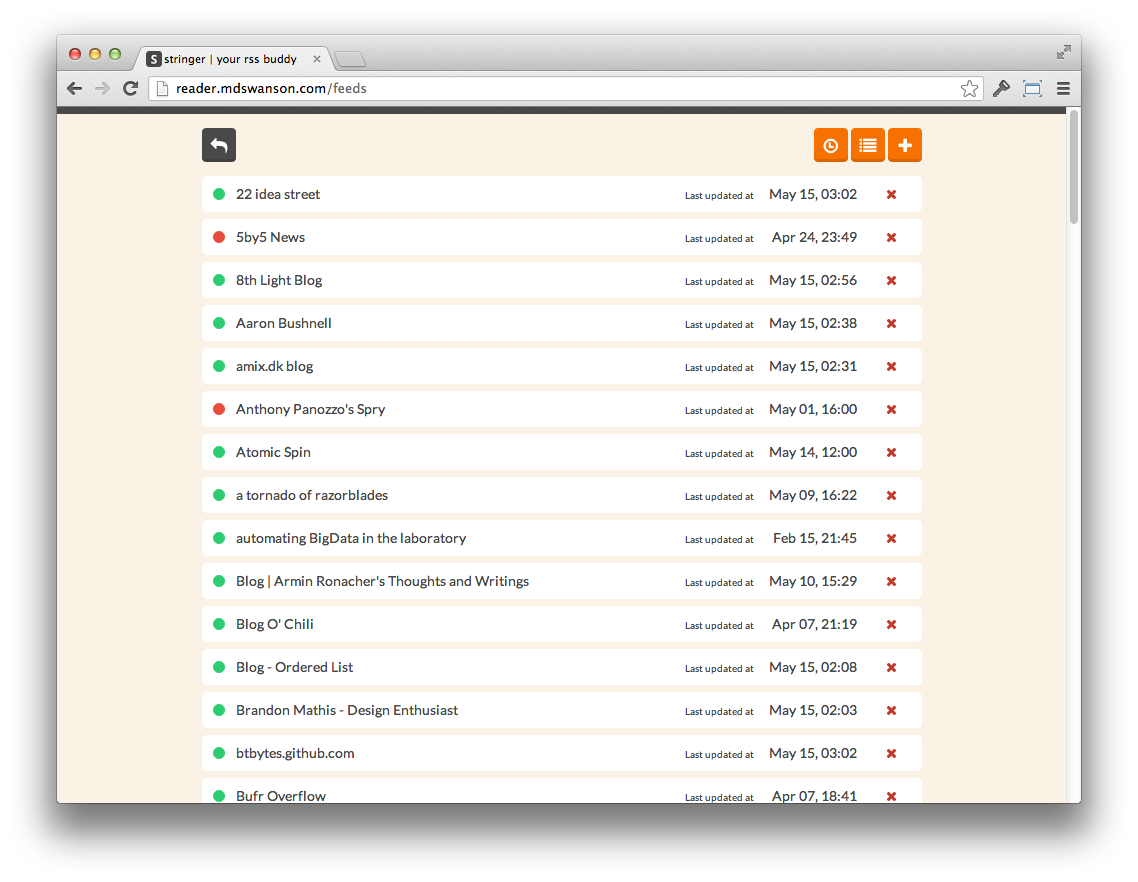This screenshot captures a website interface titled "Stringer, your RSS buddy," displayed on a browser tab. The URL in the search window reads "reader.mdswanson.com" with a section labeled "feeds." The site design features a black header strip above a creamy background, overlaid with several white slots or content blocks.

In the top-right corner, there are three distinct orange icons: a clock, a list with a yellow plus sign, and another symbol. On the top-left, there's a black key icon with a leftward arrow.

Each white slot contains a set of details, starting with a small button that indicates status—either green (active) or red (inactive). Most slots have a green button, while two have red ones. Each slot also displays a last updated time and date, followed by a red ‘X’ for deletion.

Here are the detailed contents of some slots:
1. **22 Ideal Street** - Updated May 15th at 03:02
2. **5x5 News** - Updated April 24th at 23:49 (Red button)
3. **8lightblog** - Updated May 15th at 02:56
4. **Erin Bushnell** - Updated May 15th at 02:38
5. **amx.dkblog** - Updated May 15th at 02:31
6. **Anthony Palenzo Spry** - Updated May 1st at 16:00 (Red button)
   
Additional slots visible include:
- Atomic Spin or Tornado of Razorblades
- Automated Big Data in the Laboratory
- BlogArmin
- Rancher's Thoughts and Writings
- BlogOchili
- BlogOrderless
- Brandon Mathis, Design Enthusiast
- bbbytes.github.com
- Berf Overflow

These details provide a comprehensive view of the feed updates managed within the RSS reader interface.